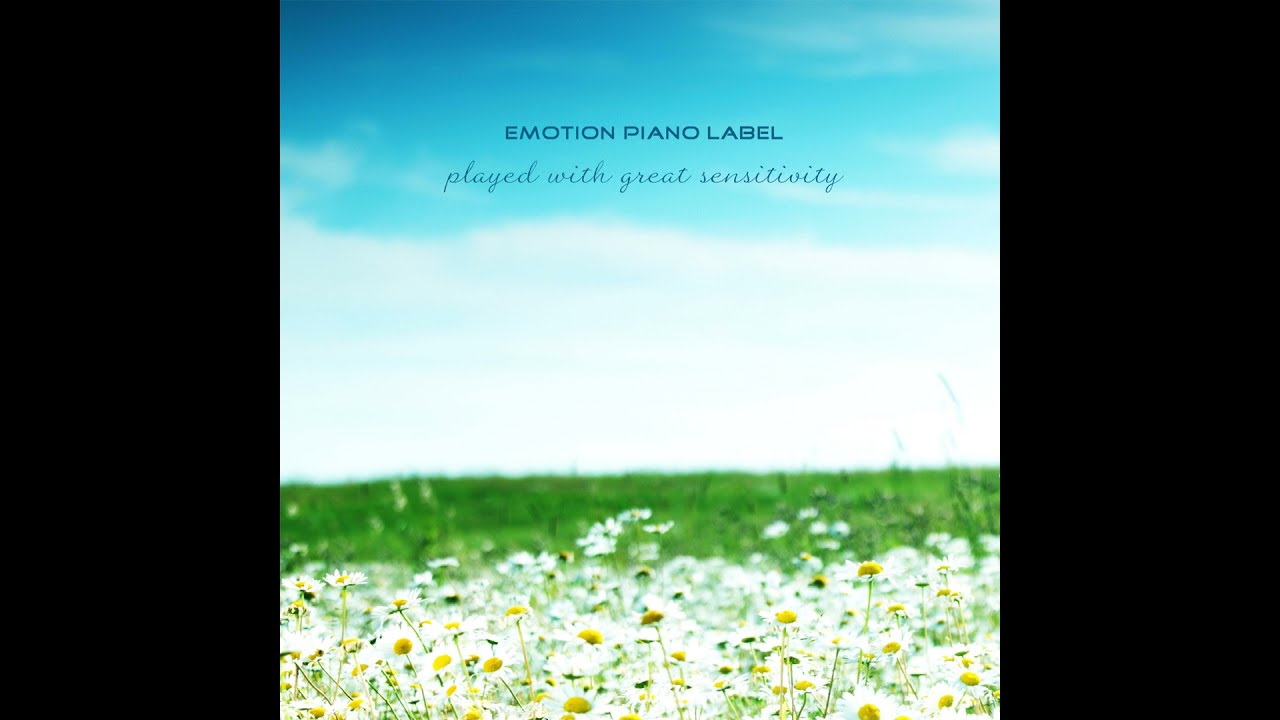The image resembles an album cover with a rectangular shape, wider than it is tall, featuring thick black borders on the left and right sides, framing a square central image. The foreground showcases a vibrant field of wildflowers with white petals and yellow centers, occupying the bottom portion of the image. Just beyond the flowers stretches an open green field. The background is dominated by a bright, sunny sky with numerous clouds on the horizon that thin out into wispy formations against a blue expanse. Centered within the top third of the image, bold block text reads "Emotion Piano Label," with the phrase "played with great sensitivity" elegantly inscribed below in cursive.